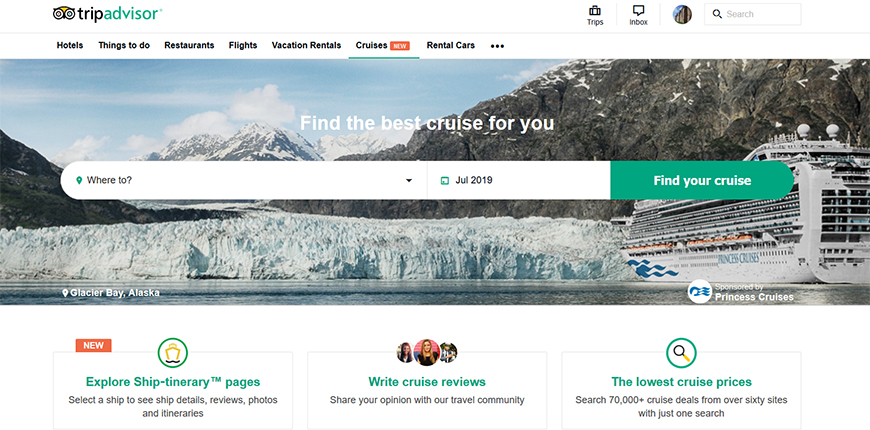The image features a predominantly white background that hosts a variety of elements indicative of a travel website, specifically TripAdvisor. At the top of the image, the TripAdvisor logo is prominently displayed, featuring the iconic owl with large, inquisitive eyes. The word "Advisor" is highlighted in green, while "Trip" is in a standard black font.

Below the logo, there's a navigation bar with options such as "Trips" and "Room," accompanied by a circular icon showing a building. Adjacent to this is a search box, hinting at the site's functionality. Further down, another white box presents various travel categories: "Hotels," "Things to Do," "Restaurants," "Flights," "Vacation Rentals," and "Cruises," the latter of which is underlined in green and tagged with a red "New" label. The categories continue with "Rental Cars," followed by an ellipsis indicating additional options.

Dominating the center of the image is a vibrant picture encapsulating a serene, picturesque scene. This image showcases a clear blue sky adorned with fluffy white clouds, towering snow-capped mountains in the background, a vast ocean, and a sizable cruise ship navigating the waters.

Just below this scenic photograph, a large search box is prominently placed. It features the prompt "Where to," accompanied by a green location pin and a downward-facing arrow for selection. Adjacent to it is another clickable box with a green calendar icon displaying "July 2019." A distinct green button labeled "Find Your Cruise" is positioned next to these elements. Below the search box, "Glacier Bay, Alaska" is mentioned with a small white location pin beside it. The phrase "Princess Cruises" is circled in blue font, emphasizing the cruise line.

In the lower section of the image, a smaller blue box is visible. To the upper left of this box, a red "New" label is displayed. A green circle featuring a ship icon and an underline is captioned "Explore Ship Itinerary Pages," inviting users to select a ship for detailed information, including reviews, photos, and itineraries.

Adjacent to this are three small circles with images of people, followed by green text that says "Write Cruise Reviews," encouraging users to share their travel experiences. The page continues with another green circle, this time containing a magnifying glass icon. The green text here reads, "The Lowest Cruise Prices," encouraging users to search over 70,000 cruise deals from more than 60 different sites in one convenient search.